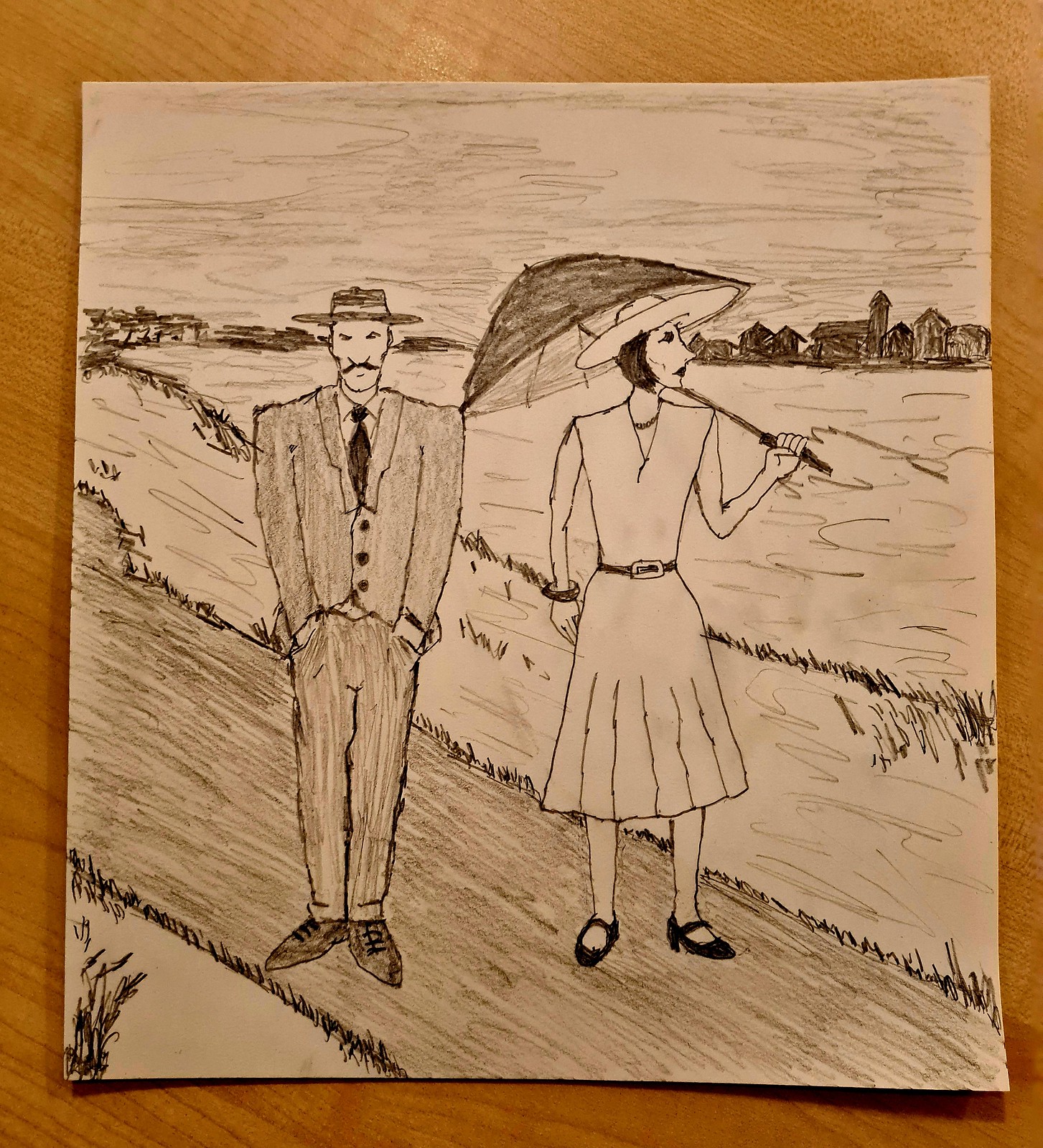This photograph captures a large, stiff white piece of paper set against a rustic maple wooden background. The lighting casts a dim, yellowish-golden glow over the entire scene, enhancing its warm and nostalgic atmosphere. On the paper is a detailed ink drawing depicting a turn-of-the-century white couple walking down a path adjacent to a body of water. The man, dressed in a three-piece suit and a hat, directs his gaze straight ahead towards the viewer. The woman, with her black hair peeping under her hat, wears a period dress and holds an umbrella over her shoulder, her attention turned towards the right side of the frame. The intricate details of their attire and the serene environment create a captivating historical snapshot.